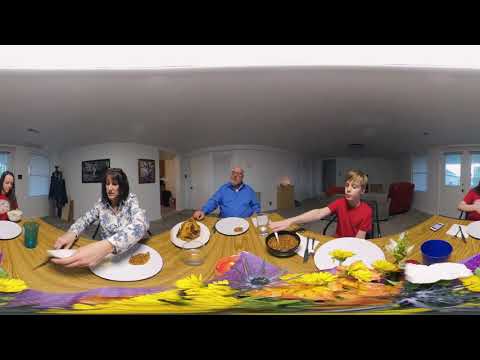The image captures a 360-degree view of a family dinner around a wooden table in a white-walled, white-ceilinged room that appears to be someone's home. The table is adorned with various foods, white plates, green glasses, blue bowls, and colorful flower decorations in yellow, purple, and pink. The atmosphere suggests a casual family gathering, with a front door visible in the background. 

Starting from the left, a girl in a red shirt with shoulder-length hair and a white bow is seated; she has an empty plate in front of her. Next to her is an older woman with shoulder-length black hair, wearing a white shirt with blue flowers. She is holding a piece of food with one hand and using a utensil with the other, with a portion of pie on her plate. 

An older man with a white beard and glasses sits to the right of the woman, dressed in a blue shirt. He has a plate with what looks like chicken or turkey in front of him, resting one hand on the table while the other is out of sight. On the man's right, a boy in a red shirt reaches into a black bowl of beans or similar food, with an empty plate beside him. The image has a slight curvature, indicative of the 360-degree perspective, creating an immersive view of the cozy family mealtime.